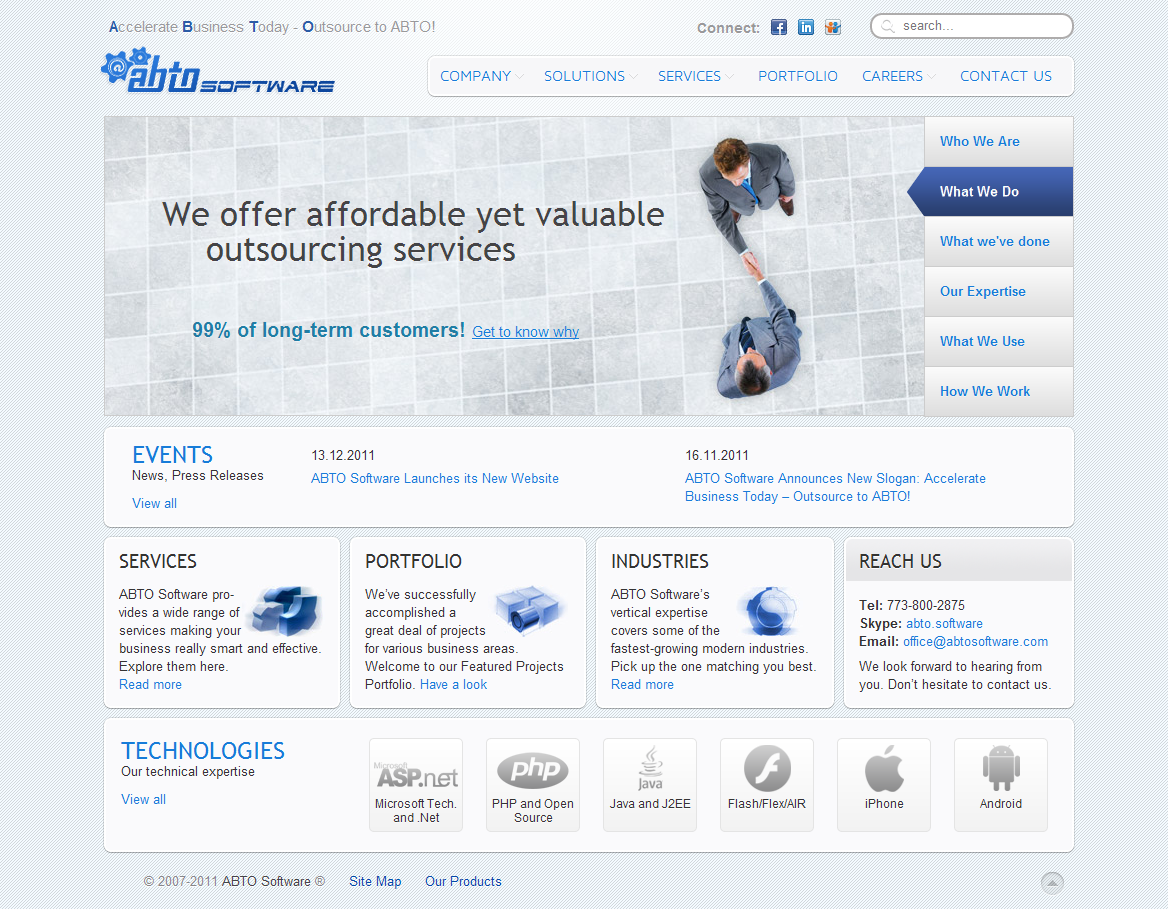OnSource ABTL Connect Launches New Business!

Today marks the launch of my new venture, OnSource ABTL Connect. Operating across platforms like Facebook and LinkedIn, our business provides innovative and affordable OnSource services to a loyal customer base, with 90% of our clients being long-term partners. We specialize in a variety of services and solutions tailored to enhance business efficiency and effectiveness.

The image captures two business professionals, both in suits, engaged in a handshake. One of them sports a blue tie and brown hair, while another figure is seen in the background, adding to the dynamic business environment depicted in the scene. The setting highlights the professional and collaborative nature of our team at OnSource ABTL Connect.

ABTL Software, integral to our service offering, covers a wide spectrum of business needs, ensuring your enterprise is smart and effective. Our portfolio showcases numerous successfully completed projects across diverse business sectors. ABTL Software is recognized for its impressive growth and speed in the industry.

For more information, visit our official website or reach out to us via telephone at 7300-275-SKY, or email us at office@abtlsoftware.com. Learn more about our services on hp.net, microsoft.com, and php webpages.

Welcome to the future of business solutions with OnSource ABTL Connect!